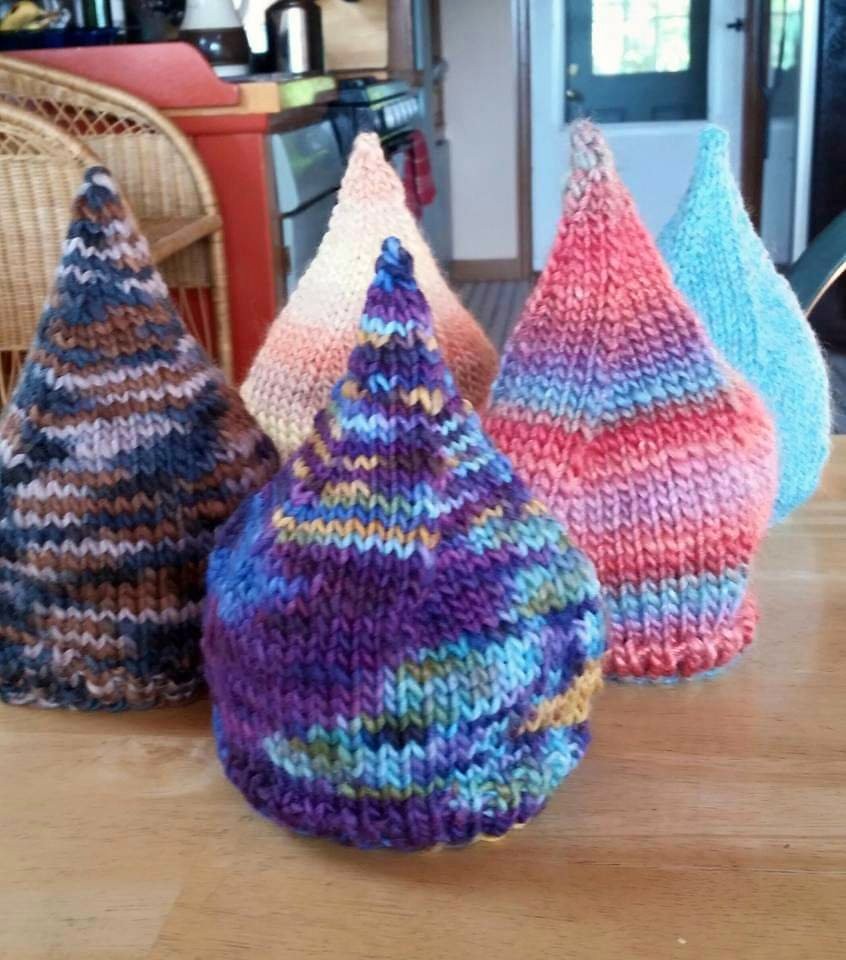The image depicts five knitted objects, resembling Hershey's Kisses or teardrops, neatly arranged on a light beige wooden surface. Each item features a rounded base with a pointed top, crafted from various types of yarn. From left to right:

1. Positioned in the back row on the left, the first object is made from yarn that blends blue, brown, and beige.
2. Next to it, also in the back row but to the right, is one with a gradient of shades ranging from peachy pink to light purple.
3. In the far right back corner, there is a bright turquoise blue object.
4. In front of the turquoise blue piece, moving towards the front, stands a vibrantly striped one featuring bright pink, purple, and blue shades.
5. The final object in the front center showcases a multi-colored design with dominant purple, blue, and green hues, and touches of yellow.

The background reveals parts of a home kitchen, including elements like a wicker basket in the upper left corner, a white door on the right, and a hint of household appliances such as a dishwasher and an oven. The flooring behind the wooden table is grayish, and the walls are a mix of beige and brown. The image captures a cozy and colorful arrangement of handcrafted fabric art against a familiar domestic setting.